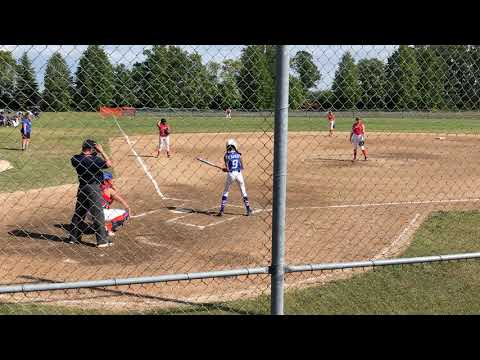The image captures an outdoor baseball game seen through a chain-link fence with prominent vertical and horizontal bars framing the shot. There are thick black borders at the top and bottom of the image. From a viewpoint just to the right of home plate, the scene reveals the batter, wearing a blue jersey with the number 9, white trousers, blue socks, and a white helmet, standing in the batter's box on sandy soil. The umpire, dressed in dark attire, stands behind the catcher to the left of the batter. On the defensive team in red jerseys, the third baseman, shortstop, and pitcher are visible, with the left fielder appearing in the far distance near the outfield fence. A coach is positioned near third base, and some spectators can be seen along the left field line. The grassy field features white boundary lines, and a row of trees delineates the background along with a visible portion of the sky.